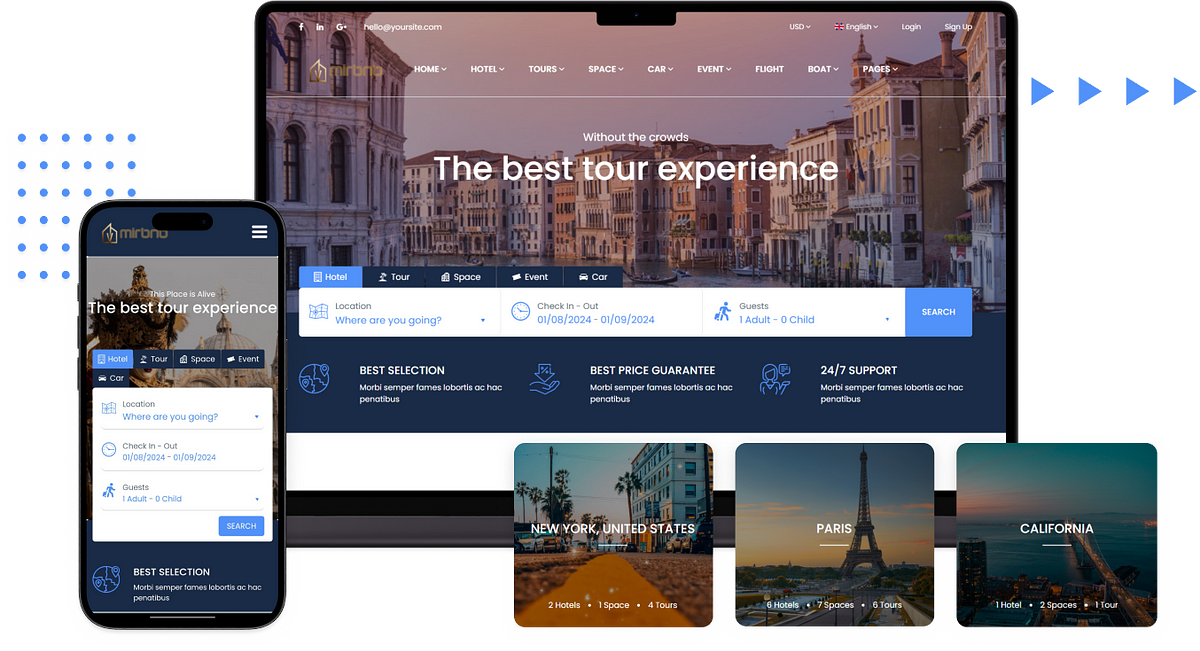Discover a comprehensive travel website offering a variety of personalized holiday trips with minimal crowds. Easily browse through three main options located at the bottom of the page: "Best Selection," "Best Price Guarantee," and "24-Hour Support." The advanced search functionality allows users to specify the number of guests, check-in and check-out times, hotel locations, and types of tours. The platform also supports car rentals, flights, and boat services, showcasing its versatility. The site, which appears to be from England, is in English and supports multiple currencies, including USD. Users can conveniently log in or sign up, and there's a dedicated mobile app available. Though it bears some resemblance to Airbnb, the exact branding is unclear.